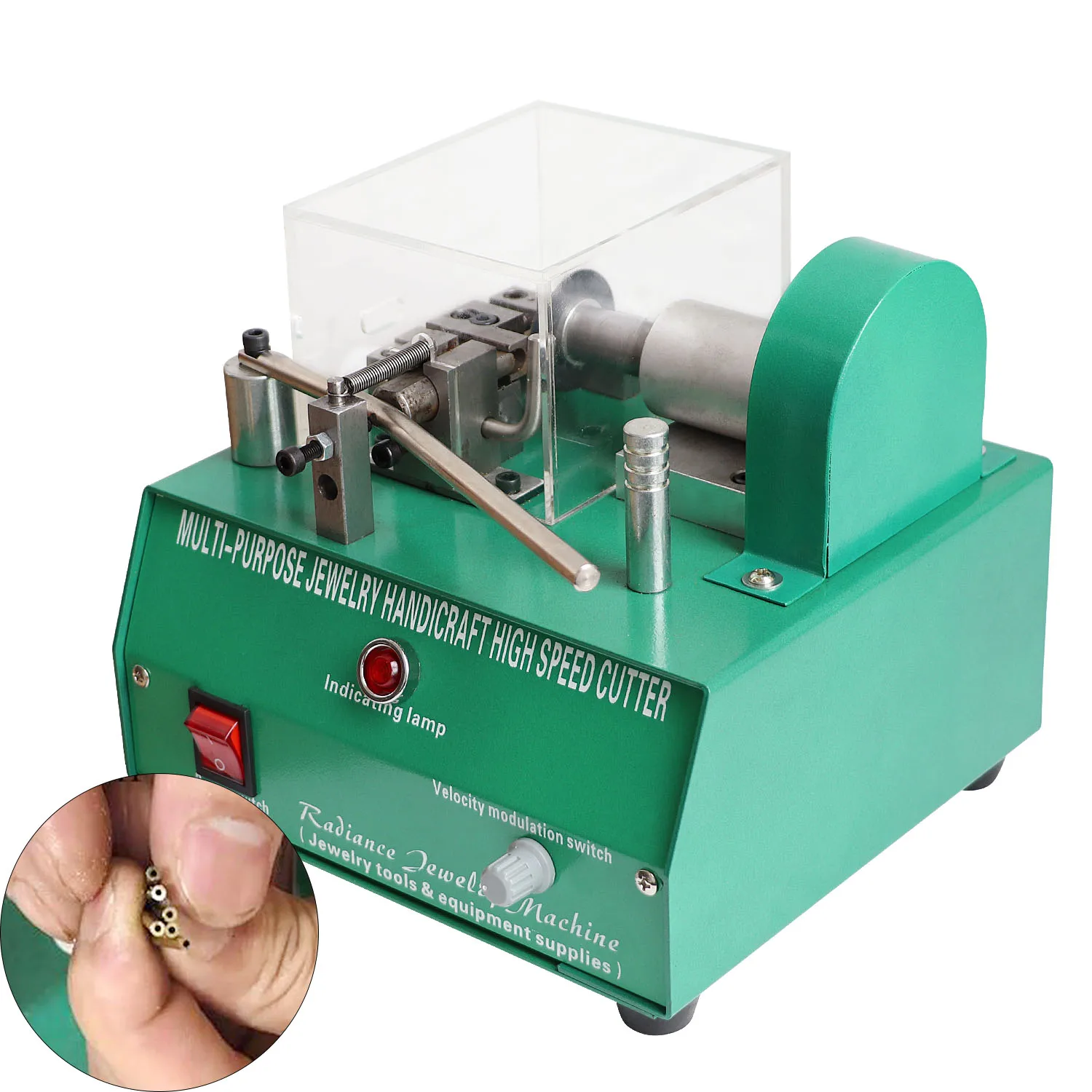The image features a teal green piece of machinery labeled as a "Multi-Purpose Jewelry Handicraft High Speed Cutter." The front face of the machine prominently displays this label along with the term "Radiance Jewelry Machine - Jewelry Tools and Equipment Supplies." The machine is diagonally oriented, with various controls and indicators on its front. A red power switch is located on the lower left, accompanied by a velocity modulation knob to its right, which regulates the speed. Below the main label, there's a red indicating lamp that lights up during operation. The device also has a fuse cover on the top right.

The cutting mechanism is housed under a small plastic cover, designed to keep dust and debris contained. Inset in the photo is a close-up of fingers holding several small, hollow metal tubes, depicting the type of delicate items the tool is intended to cut. Additional visible components include a wheel and various metal parts essential to the machine's operation.